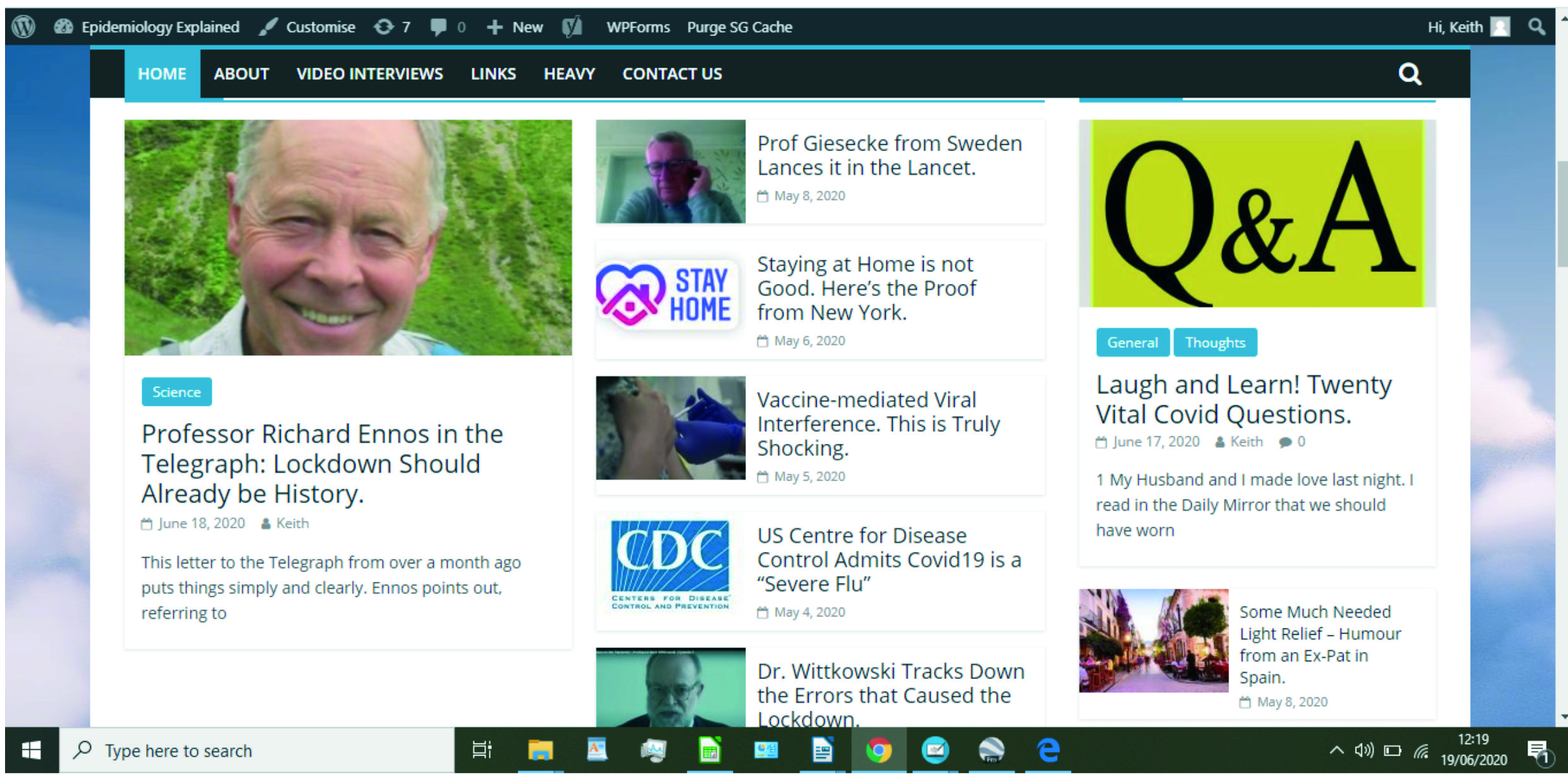**Detailed Caption:**

This is a screenshot of a medical-related website that features various articles and elements pertinent to the COVID-19 pandemic. 

Starting from the top left corner, there is a picture of a middle-aged man smiling at the camera, alongside a headline that reads, "Science." This section highlights an article titled, "Lockdown Should Already Be History," by Professor Richard Anos, published in The Telegraph on June 18, 2020. The article, a letter from over a month ago, succinctly explains Anos' viewpoints on the lockdown's necessity and timing.

In the middle column, another photo features a man wearing glasses, identified as Professor Giesecke from Sweden. This section references his piece in The Lancet, featuring an icon of a heart inside a house with the message, "Stay Home." The headline under this icon reads, "Staying at home is not good. Here's the proof from New York," indicating a critical examination of home isolation policies.

Further down, there is an image of a person receiving an injection in the arm, accompanied by the caption, "Vaccine-Mediated Viral Interference," referring to some shocking findings in the article. An adjacent icon with the letters "CDC" denotes the U.S. Center for Disease Control, followed by a headline declaring, "COVID-19 is a severe flu," reflecting a controversial admission.

Below this, a photograph of a man in glasses introduces Dr. Wachowski, who "tracks down the errors that caused the lockdown," indicating an analytical piece on lockdown missteps.

On the far right side of the page, a rectangle with a greenish background contains a clickable Q&A section with the headline, "Laugh and Learn: 20 Vital COVID Questions." Beneath this, a photograph of a city street is captioned, "Some Much-Needed Light Relief," sharing humor from an expatriate in Spain to lighten the otherwise serious tone of the website content.

Through a combination of imagery and text, the website aims to offer diverse perspectives on the COVID-19 pandemic and its management, featuring articles from notable experts and reflective pieces on global responses.